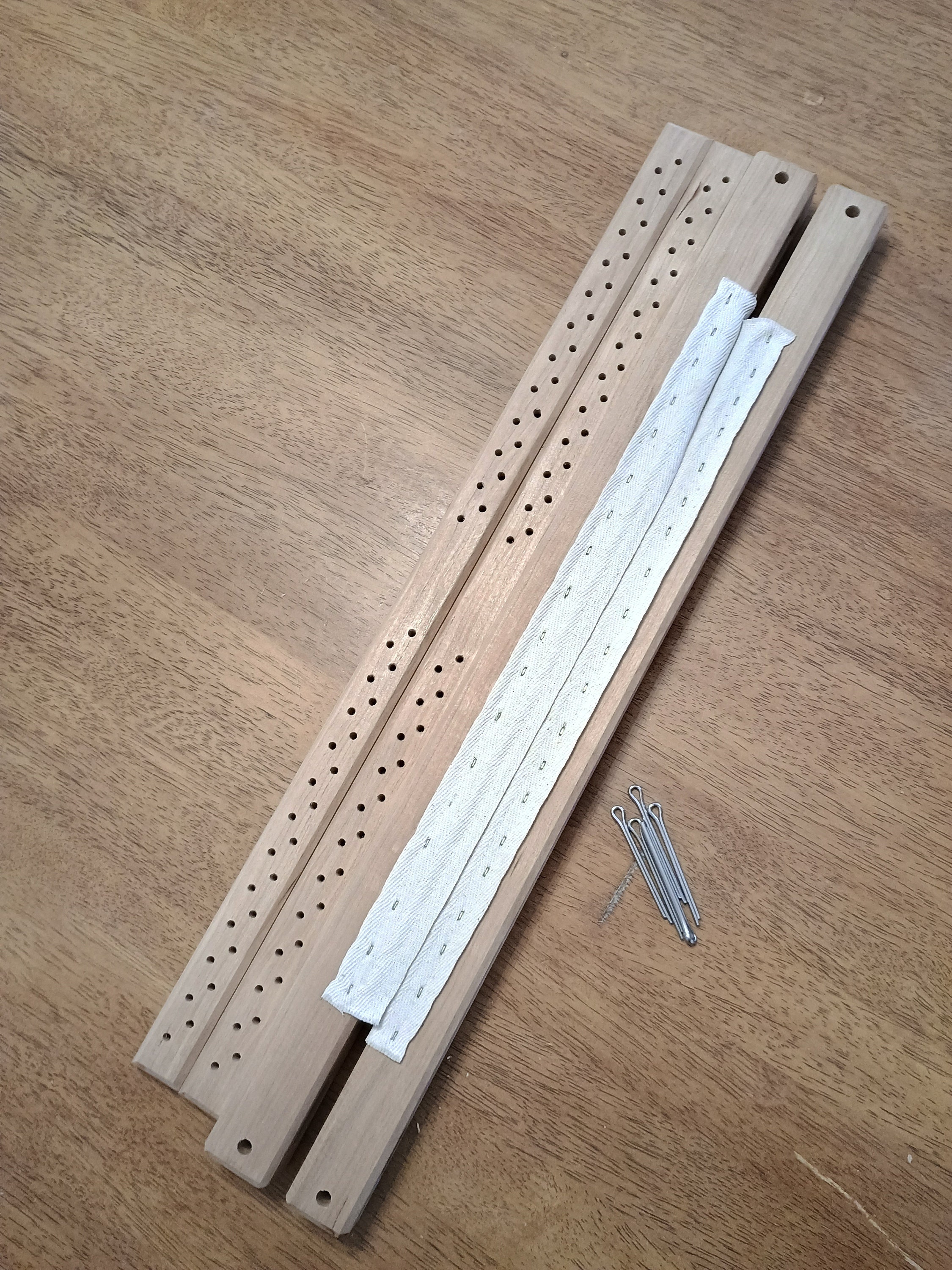The image features four wooden pieces arranged diagonally on a light brown wooden table. The two pieces on the left are distinguished by numerous small perforated holes, while the two pieces on the right each have a single hole close to their ends, making a total of two holes per piece. These right-hand pieces also have sections of thin white fabric stapled onto them. Next to the wooden pieces are four silver-colored metal clips, one of which has a slightly looped end. The table has a noticeable light brown burn mark underneath the wooden clips and a droplet stain above them. The wood appears new, possibly freshly cut, and the components seem to fit together purposefully, though no diagram is provided to explain their assembly.